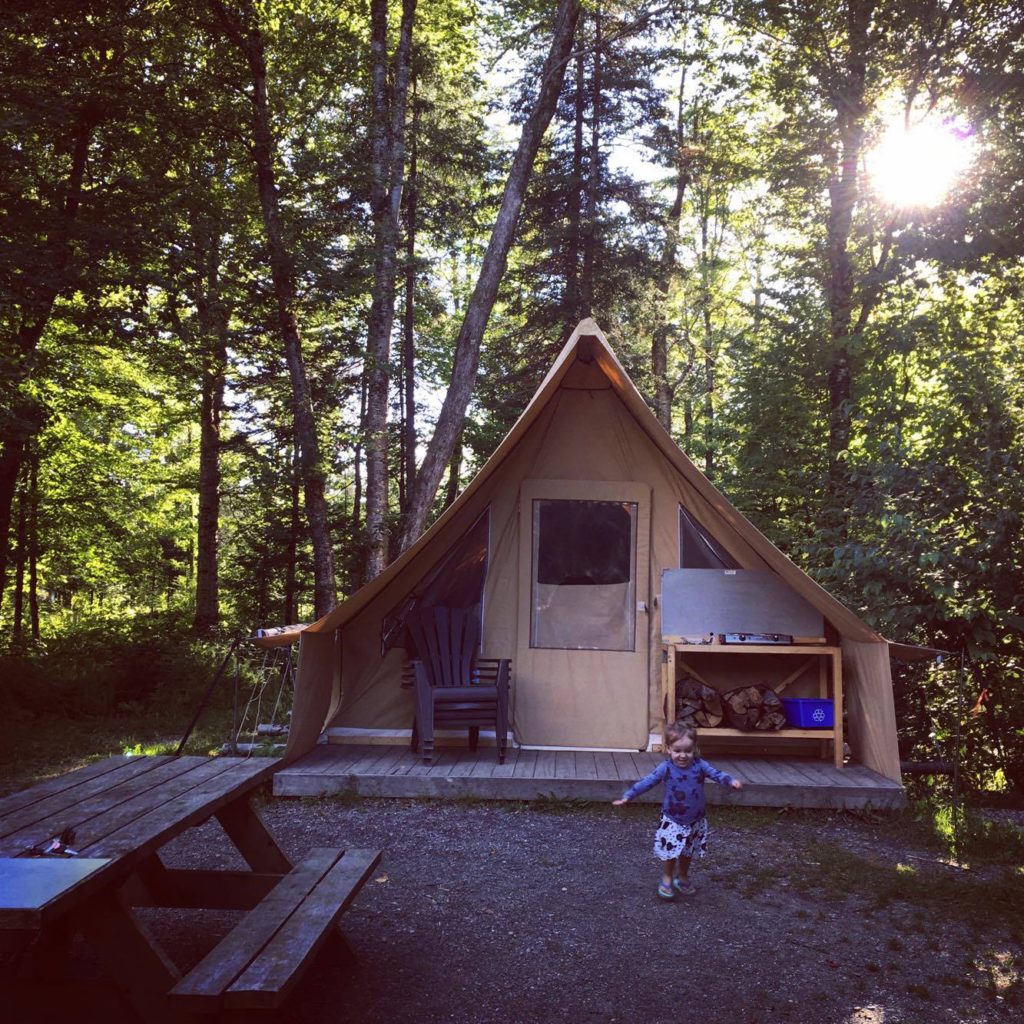On a bright, sunny summer day under a clear blue sky, a quaint tent-like cabin, reminiscent of a small A-frame house, stands amidst a forest with varied trees. The cabin, situated on a wooden platform that extends to form a porch, features a door flanked by a stack of dark-colored plastic chairs on one side and a makeshift wooden shelving unit on the other. The shelving holds logs of cut wood and a blue plastic box, possibly a recycling bin, with a table resting atop it.

In front of the cabin, where the wooden planks meet the ground, patches of dirt and grass create a rustic feel. A wooden picnic table, partially laden with what looks like a set of keys and a cutting board, sits to the left. A joyful toddler with brown hair, a blue and black shirt, a white and black print skirt, and flip-flops runs gleefully on the grass. The child’s arms are outstretched as she enjoys the carefree summer day.

The entire scene is enveloped by the forest, with thin trees allowing glimpses of the high sun, emphasizing the serene beauty of this potential campground or vacation rental spot.